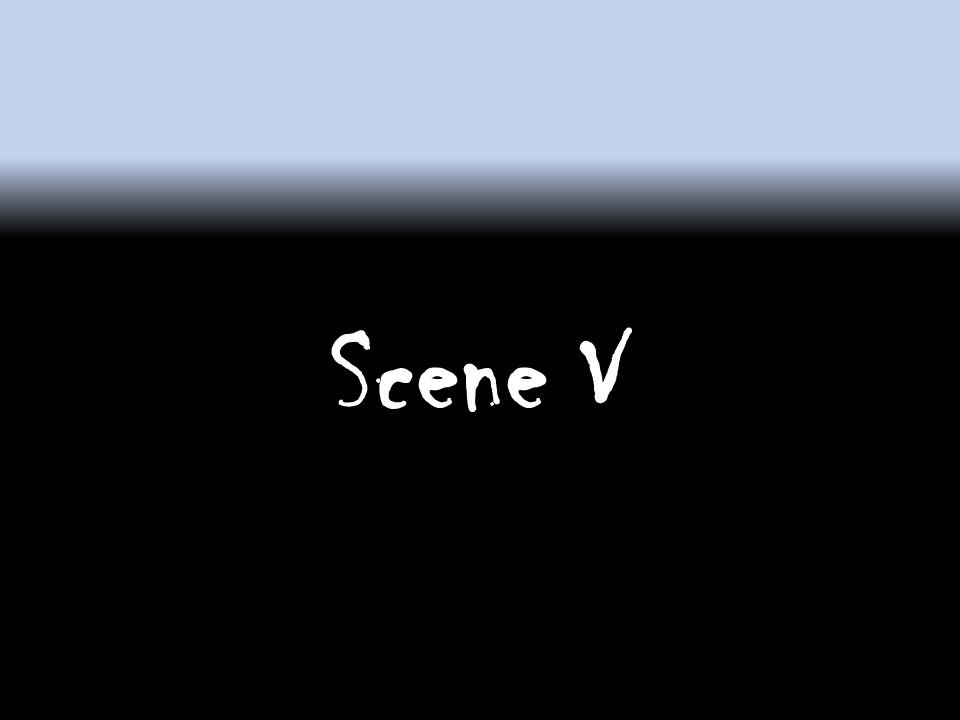The image is a basic scene card with a gradient background blending from a bluish-purple top section to a predominantly black bottom section. The background features a blue banner running horizontally at the top, which transitions smoothly into the black, creating a grayish blend where the colors meet. The black background takes up approximately 80% of the image, with the top bluish-gray portion comprising the remaining 20%. In the center of the black section, the text "SCENE V," written in white, is prominently displayed. This text appears to use a hand-painted style, evident in the varying thickness of the strokes—particularly noticeable on the 'S' and 'N', where the paint seems to taper off towards the bottom. Additionally, there are small white paint dots near the 'N' and 'C'. Overall, the image features a simplistic design, likely intended as a transition slide for a low-budget movie, with no other objects present.